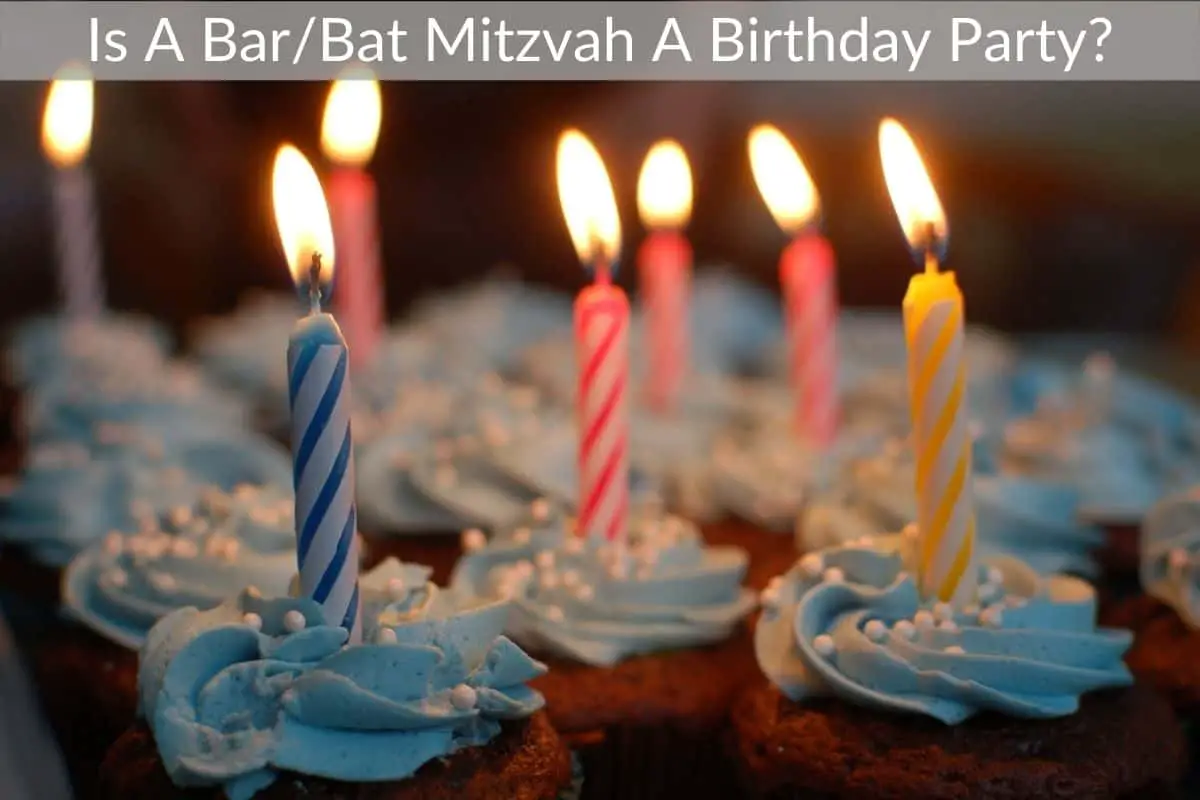This is a close-up photograph of approximately 15 dark brown chocolate cupcakes decorated for a special occasion. Each cupcake is adorned with a light blue frosting sprinkled with small yellow circles. Upright in the frosting, there are various lit candles, including blue and white striped, yellow and white striped, pink and white striped, and a few candles in the background with distinct colors such as purple. 

At the top of the image, there is a horizontal, translucent gray bar with bold white text reading: "Is a bar/bat mitzvah a birthday party?". The entire scene appears to be set indoors in a dimly lit room, enhancing the warm glow of the candle flames and emphasizing the celebratory atmosphere.